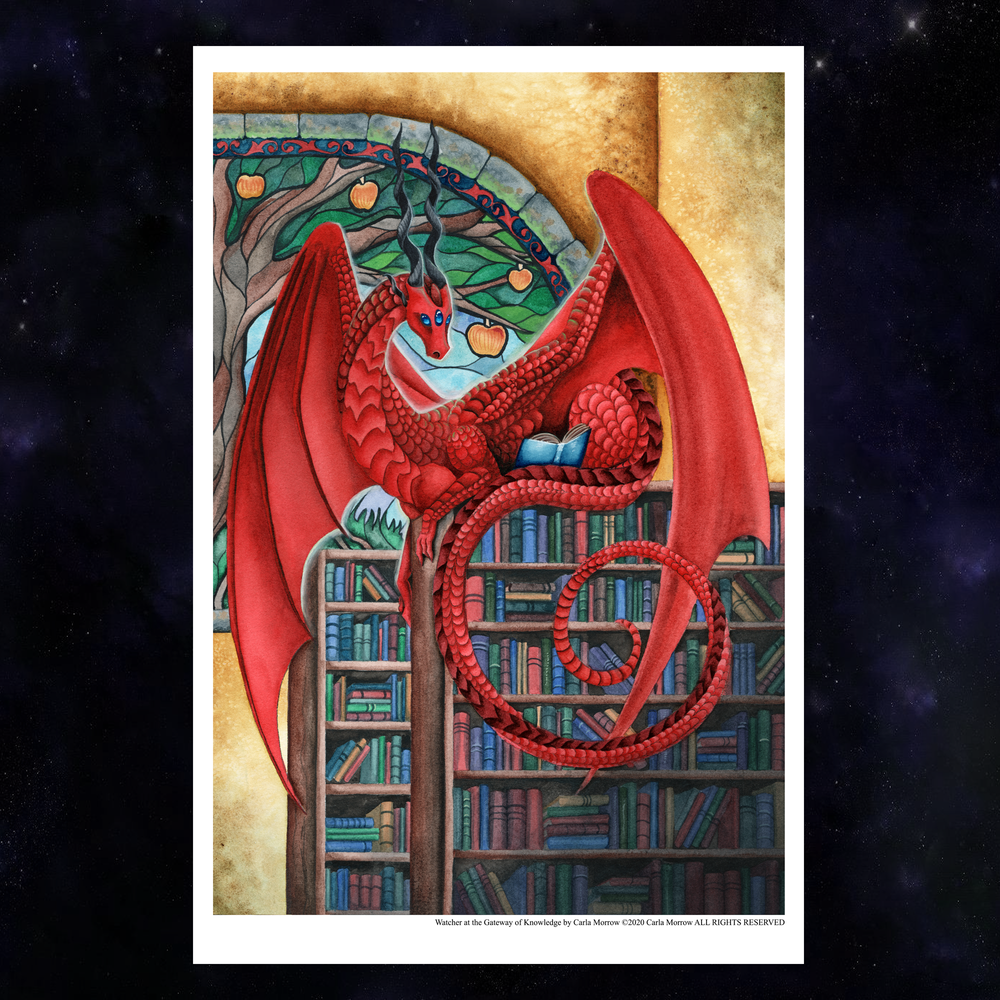The image is a vibrant illustration featuring a majestic red dragon perched atop a well-stocked bookcase. The scene is animated and framed by a simple, white, square-shaped border. The lower right corner of the image contains a small, nearly illegible series of black text. The front-view bookcase showcases an array of colorful books with spines in hues of red, blue, orange, green, and brown. Dominating the scene, the red dragon’s body is positioned with an elegant, swirling tail at the base, and its expansive red wings extended. The background wall behind the bookcase is a soft light brown, and a cutout window reveals a lush tree adorned with green leaves and plump orange apples. The outer backdrop of the image features a captivating galaxy-like theme, predominantly black with enchanting splashes of purple.